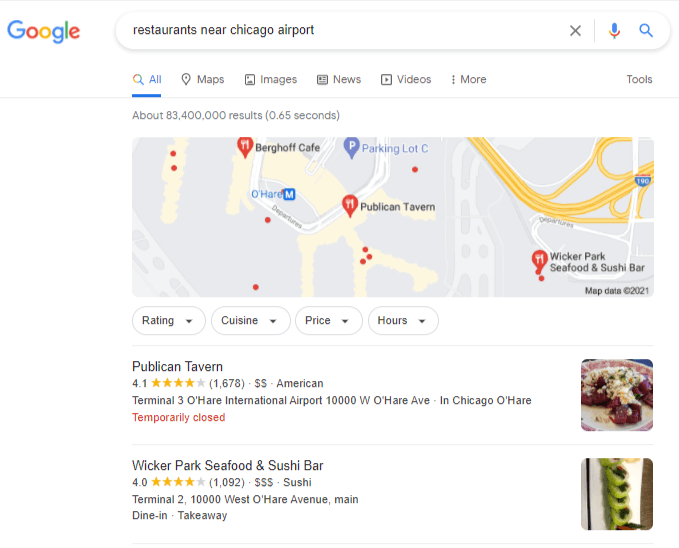The image depicts a desktop screenshot showcasing a Google search related to finding restaurants near Chicago airport. The user has typed "restaurants near Chicago airport" into the search bar. The familiar icons are present, including the 'X' to clear the search, the microphone for voice search, and the magnifying glass to initiate the search. Adjacent to these is the locator pin for maps, followed by options for images, news, videos, more, and tools.

The search yielded approximately 83,400,000 results within 0.65 seconds. Displayed prominently is a map highlighting different restaurant locations around the Chicago O'Hare International Airport. 

Two restaurants are specifically noted. The first one, Publican Tavern, holds a rating of 4.1 stars from 1,678 reviews. This American-style eatery, described as somewhat pricey, is located within Terminal 3 at O'Hare International Airport, 1010000 West O'Hare Avenue, Chicago. However, it is temporarily closed. The image associated with Publican Tavern showcases some food items.

The second highlighted restaurant is Wicker Park Seafood and Sushi Bar, rated 4 stars based on 1,092 reviews. Known for its high-priced sushi offerings, it sits in Terminal 2 at 10000 West O'Hare Avenue, Chicago. The services available include dine-in and takeaway, accompanied by an image illustrating their sushi dishes.

Additionally, the map includes another restaurant, Berghof Cafe, though no specific details about this establishment are provided in the screenshot.

In summary, the search results indicate an exploration of dining options near Chicago O'Hare International Airport, with detailed information available for two on-site restaurants.